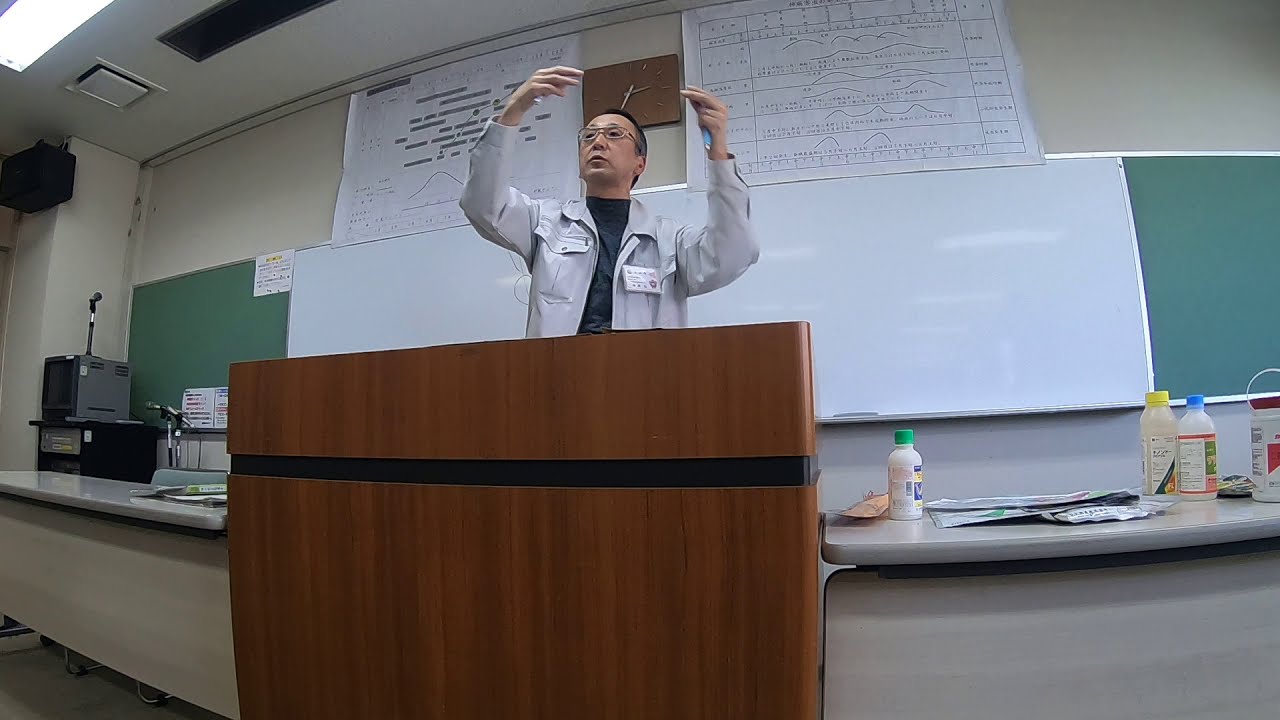The photograph captures a detailed classroom scene. Dominating the back wall is a large, long whiteboard, flanked by two green blackboards. Above these, the top part of the wall is painted white and features a brown clock positioned between two large sheets of paper displaying graphs with Asian writing. In the foreground, two long desks bracket a wooden platform from which a professor teaches. The professor, an older Asian man wearing a black shirt under a white lab coat adorned with a badge on his chest pocket, stands with arms outstretched, gesturing animatedly. He wears regular glasses and appears to be deeply engaged in his lecture. To the left of the platform, a microphone set up suggests the classroom may be used for presentations or lectures, possibly at the college level. The presence of various school materials, potentially including chemistry supplies, reinforces the academic atmosphere of the room.